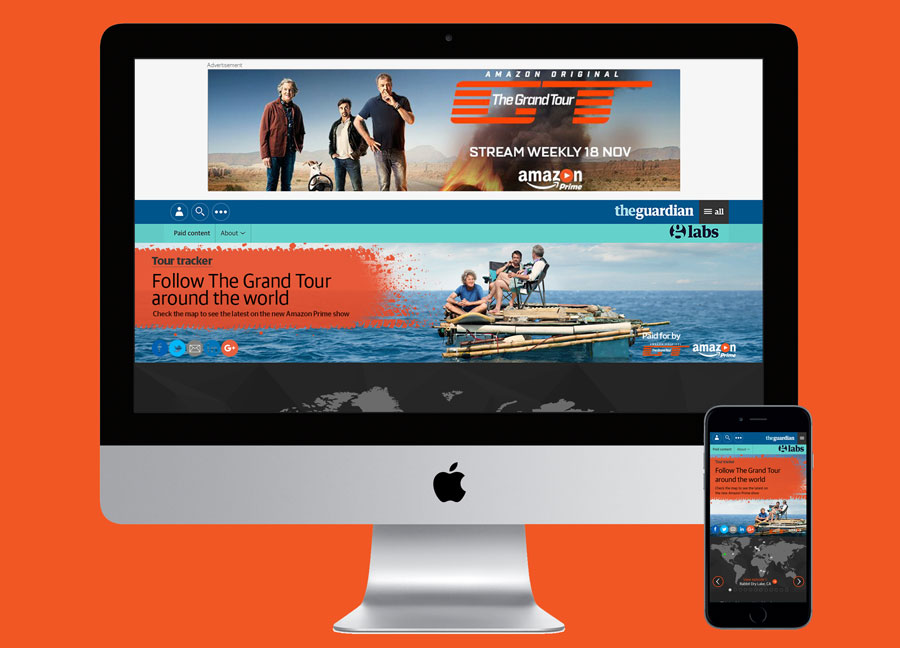The image features an Apple computer monitor with a distinctive orange background. The monitor is supported by a sleek gray stand, and the bottom bezel of the screen is also gray, adorned with a black Apple logo prominently at the center. Above the logo, the display area is primarily black, with a black border that extends around the top and sides of the screen.

At the top of the screen, there is an advertisement banner that reads, "Amazon Original The Grand Tour. Stream Weekly 18 November on Amazon Prime." The ad showcases a picturesque desert landscape with three men standing and looking directly at the camera.

Beneath this, there is a blue banner labeled "The Guardian" that includes an image of people on a fishing boat set against a light blue sky. The text on the banner mentions, "Tour Tracker: Follow The Grand Tour Around the World," with additional text that is unfortunately too small to read clearly.

Additionally, a smartphone is positioned at the bottom right corner of the monitor. The phone's screen displays the same image of the men on the fishing boat, as well as a portion of a world map directly below the image.